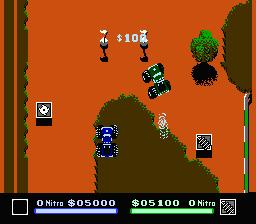This image appears to be a low-resolution, pixelated screenshot from an old video game, likely from the 90s, reminiscent of Game Boy or early computer games. The image has a top-down perspective with simple 3D elements, dominated by a predominantly red background, and various brown patches, possibly representing dirt tracks. 

At the center of the image are two vehicles: a dark blue car and a green car, suggesting a racing scenario. The cars seem to be heading towards what appears to be a finish line, indicated by two posts with white flags. Near the top right corner, there’s a small tree, adding to the rudimentary scenery.

The bottom of the screen features a black status bar extending the entire length, with distinct sections for game stats. On the left side of the bar, there is a mauve (incorrectly referenced as blue) section labeled “Nitro,” and a dollar sign followed by “050000.” On the right side, a green section shows another “Nitro” label and a dollar sign with “051000,” indicating a score or currency total of $5,100 for the green car. Overall, the image depicts a simple, nostalgic racing game interface with clear numerical performance indicators.